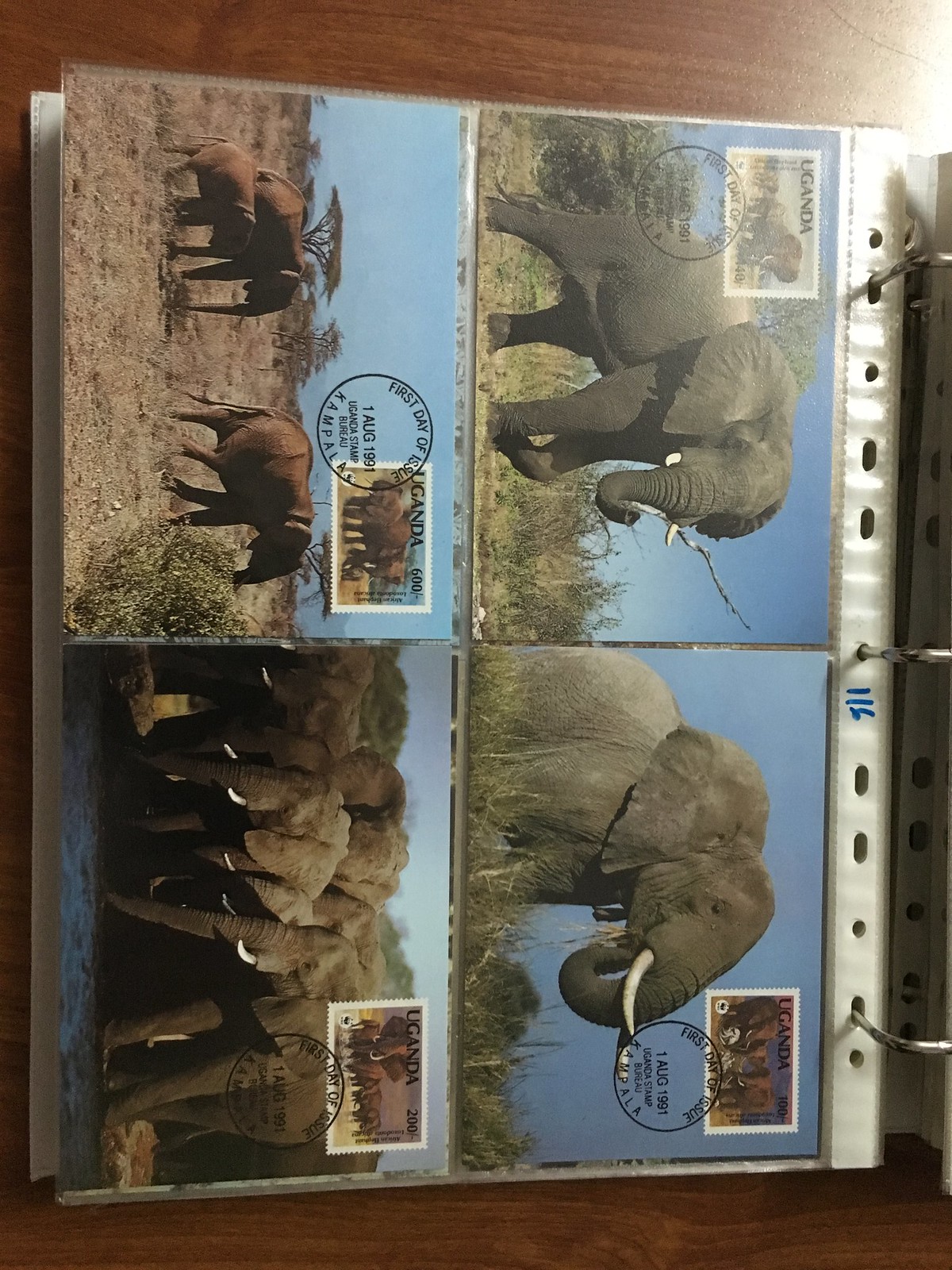The image depicts an open page of a three-ring binder resting on a wooden surface, viewed from the side. The page contains a plastic sleeve with four inserts, each holding a postcard. These postcards are protected by plastic covers and feature various images of grey elephants taken in different angles and groupings, showcasing the diverse landscape of Africa, particularly the Serengeti, with its distinct trees and pale blue skies. Each postcard is stamped with a Ugandan stamp, dated "First Day of Issue 1 AUG 1991," showcasing intricate stamp designs. The binder rings are visible on the right-hand side, securing the page in place. One postcard notably shows an elephant eating, while another depicts an elephant holding a stick. All the postcards are from Uganda, marked by their official stamps and the date of issue, reflecting a collection that captures the essence of African wildlife.